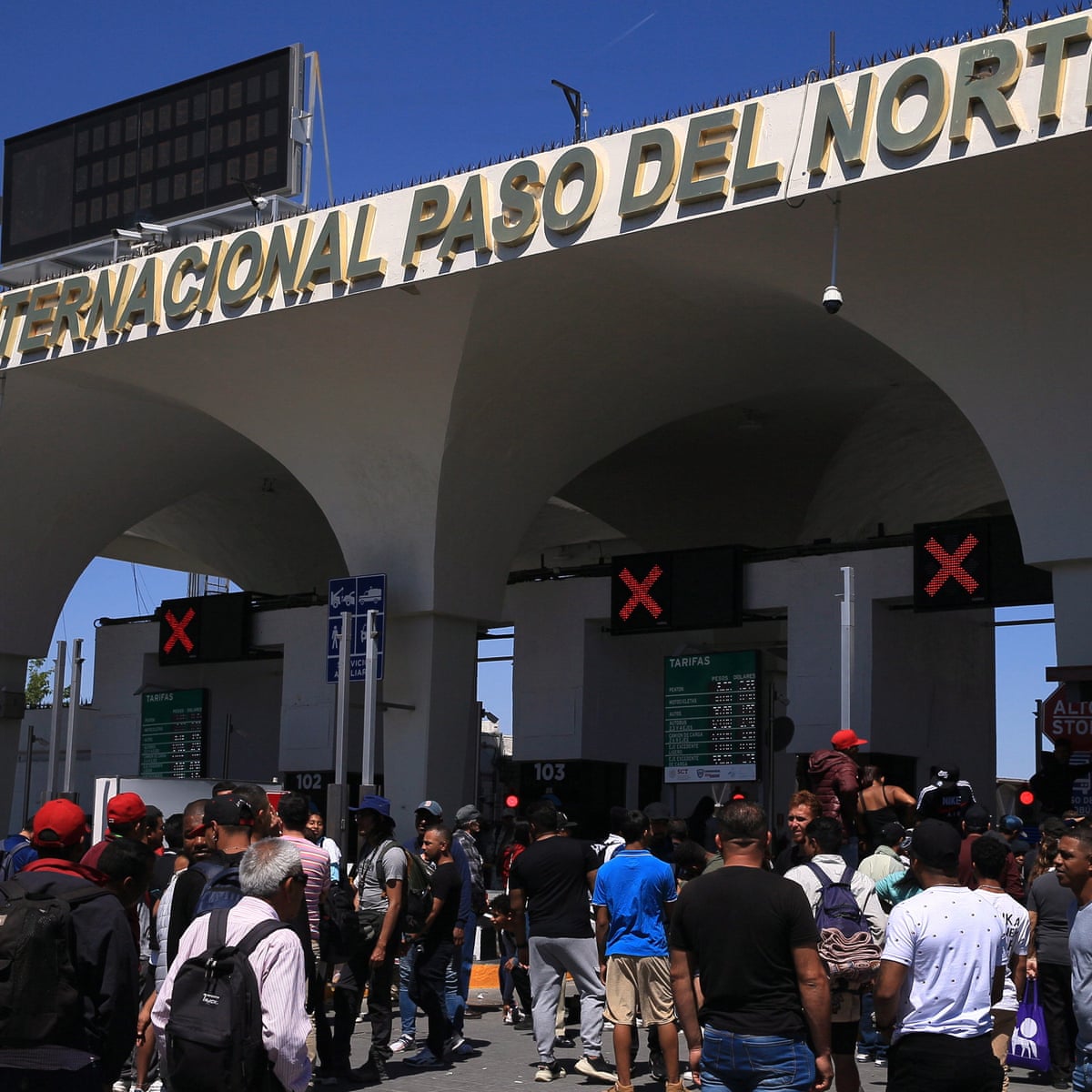The image depicts a bustling outdoor transportation station, likely an international travel checkpoint, characterized by its striking architectural features and numerous people. The prominent structure features super tall, white, curved archways, supported by gray pillars, casting shadows below. Above the structure, in bold stainless steel letters against a white background, is the inscription "International Paso del Norte," partially obscured but indicative of a crossing or border facility. Black signs featuring large red X's are prominent above the entrances, indicating stoppage or control points.

A diverse crowd is gathered below, including men and women of various ages, many wearing hats and backpacks. Among the crowd, key details include individuals dressed in varied attire such as a man in a blue shirt and light brown shorts, another in a black shirt and blue pants, and one in a white T-shirt with black pants. Some people appear to be in motion, walking towards the structure, while others mill around, creating a dynamic, lively scene.

The backdrop showcases a vividly dark blue sky, enhancing the contrast with the light-colored archways. Additional structural elements include lit panels under the archways and vertical pipes on the left side of the image, adding to the industrial aesthetic. The ground is a neutral gray, complementing the subdued tones of the pillars and providing a stark canvas for the bustling human activity.